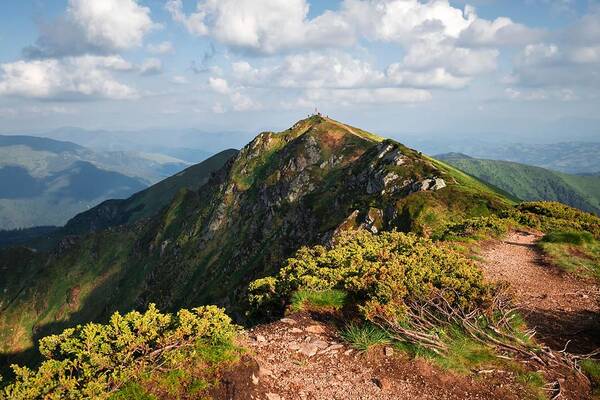In this photo, we're treated to a breathtaking view from a high vantage point, looking out over a mountainous landscape. In the foreground, the ground is predominantly dirt, interspersed with patches of grass and clumps of bushes, some of which look almost like stacked twigs and branches. To the left, the terrain drops off sharply at the cliffside. The focal mountain in the distance is draped in lush green foliage, with occasional rocky outcrops peeking through the cover of grass. Behind this main peak, two more mountain ranges stretch out towards the horizon, slightly out of focus but similarly covered in green vegetation. The sky above is a medium blue, adorned with a scattering of thick white clouds, characterized by their flat bottoms and fluffy, mound-like tops. This serene and picturesque scene is captured from a high vantage point, enhancing the depth and grandeur of the mountainous expanse.